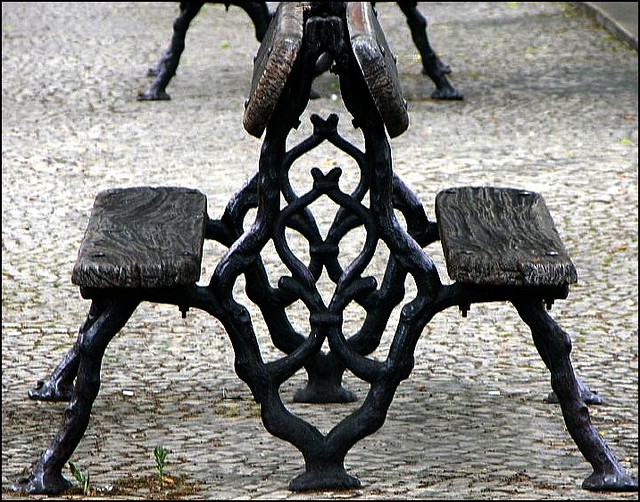The image showcases two intricately designed outdoor benches set against a cobblestone ground with small green plants sprouting in between the stones. The benches, which are positioned back-to-back, feature seats that are either dark grey metal with a wooden appearance or actual wood treated to appear shiny and weathered. This material gives off a dark brown, almost black finish. The benches are supported by an artistic black metal frame resembling jagged tree branches or flame-like diamond patterns that seamlessly connect the seats. The unique design is carried throughout the frame, giving the benches a striking, sculptural quality. In the background, additional benches of the same style are visible, emphasizing the cohesive aesthetic. The ground beneath is primarily cobblestone with a light brown tone, interspersed with patches of greenery and a small gray concrete sidewalk in the top right of the frame. Notably, there is a single cigarette visible in the bottom left corner of the image.